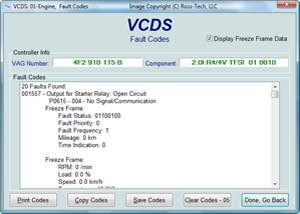The image is a very small, horizontal screenshot of a computer window, seemingly from an older version of Windows, possibly Windows XP. The window appears to be part of a program by Rosatec LLC, titled "VCDS - Fault Codes" in blue/navy text at the top. The window is framed by a light blue border and contains a white box with text. Near the top, there is a VAG number displayed in green text and some component information containing a mix of numbers and letters. This section is labeled with "VAG number" and "Component". The main text box below them includes technical details, such as fault priority and fault frequency, with various numerical values. A slider bar on the right side allows navigation within the text box. Five buttons line the bottom of the dialog box, labeled "Print Codes", "Copy Codes", "Save Codes", "Clear Codes", and a fifth option that could be "Done, Go back" or "06".